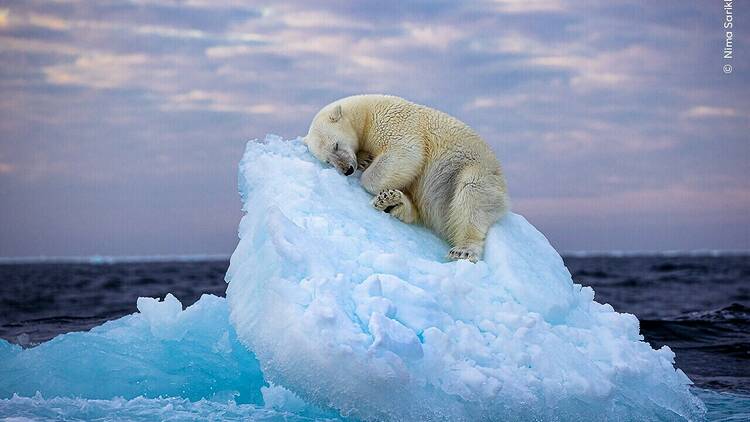A serene and picturesque scene captures a lone polar bear peacefully resting on an angled ice slab in the ocean. The bear, with its white fur, lies comfortably on its right side, offering a clear view of its left profile. Its front legs are crossed over its chest while its hind legs are positioned distinctly—with the left leg resting flat and the right leg raised, exposing its paw. The ice slab is positioned at approximately a 45-degree angle, appearing slightly elevated and seemingly floating above the deep blue, nearly black water that shows a few gentle waves. The sky above transitions to night, colored in a periwinkle hue with light clouds drifting across, enhancing the tranquil, natural setting. The overall atmosphere exudes a sense of untouched wilderness, akin to a follow-up shot from the iconic Coca-Cola polar bear commercials, capturing the bear in its undisturbed slumber amidst a breathtaking, icy expanse.